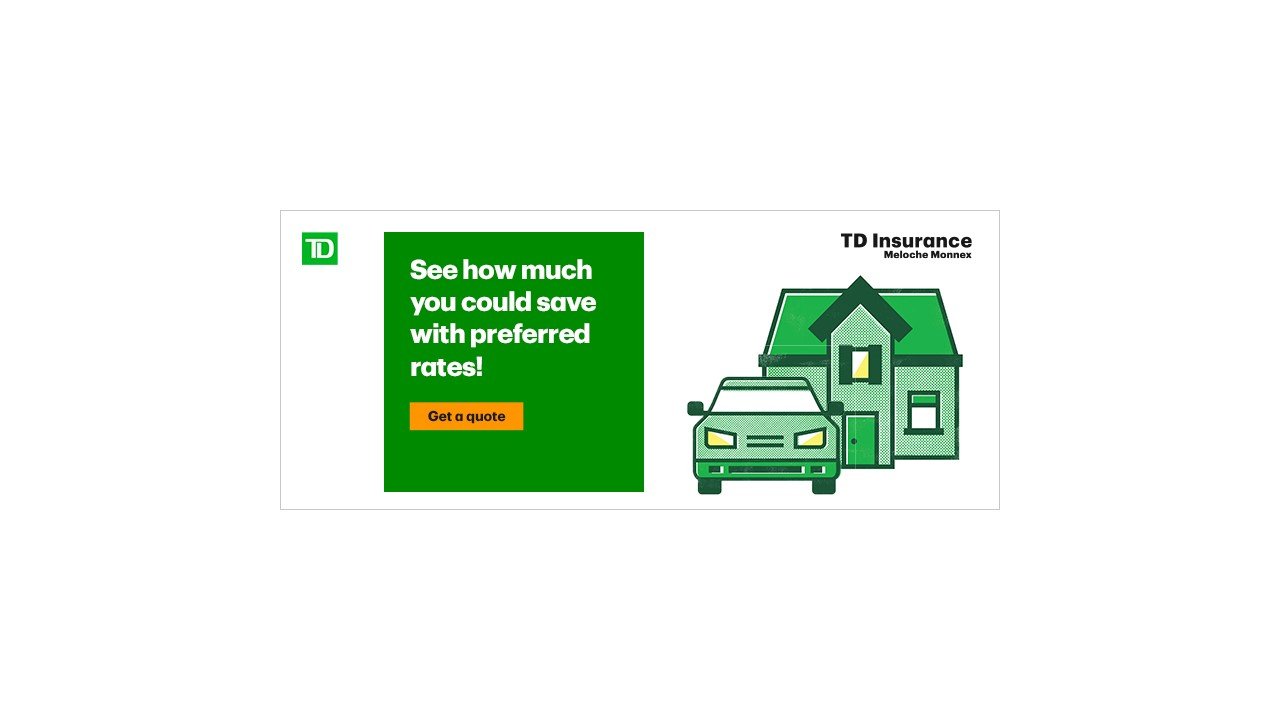This is a small, rectangular, horizontal image. In the upper left corner, there is a small green square with the white text "TD," indicating TD Bank. To the right of this is a larger green rectangle that spans nearly the entire length of the image. Inside this green rectangle, in white font, it reads, "See how much you could save with preferred rates." Below this text, within the green rectangle, there is a yellow button labeled "Get a Quote." 

Next to the green rectangle, there is a simple, icon-like graphic of a car parked in front of a house, utilizing only blue and green colors. Above the house, in the upper right corner, "TD Insurance" is written in black text. Beneath that, in very small letters, is the text "M-A-L-I-O-C-H-E M-A-N-N-E-S," although this part is somewhat unclear and difficult to read. The overall design is minimalistic and straightforward, featuring simple computer-generated graphics.